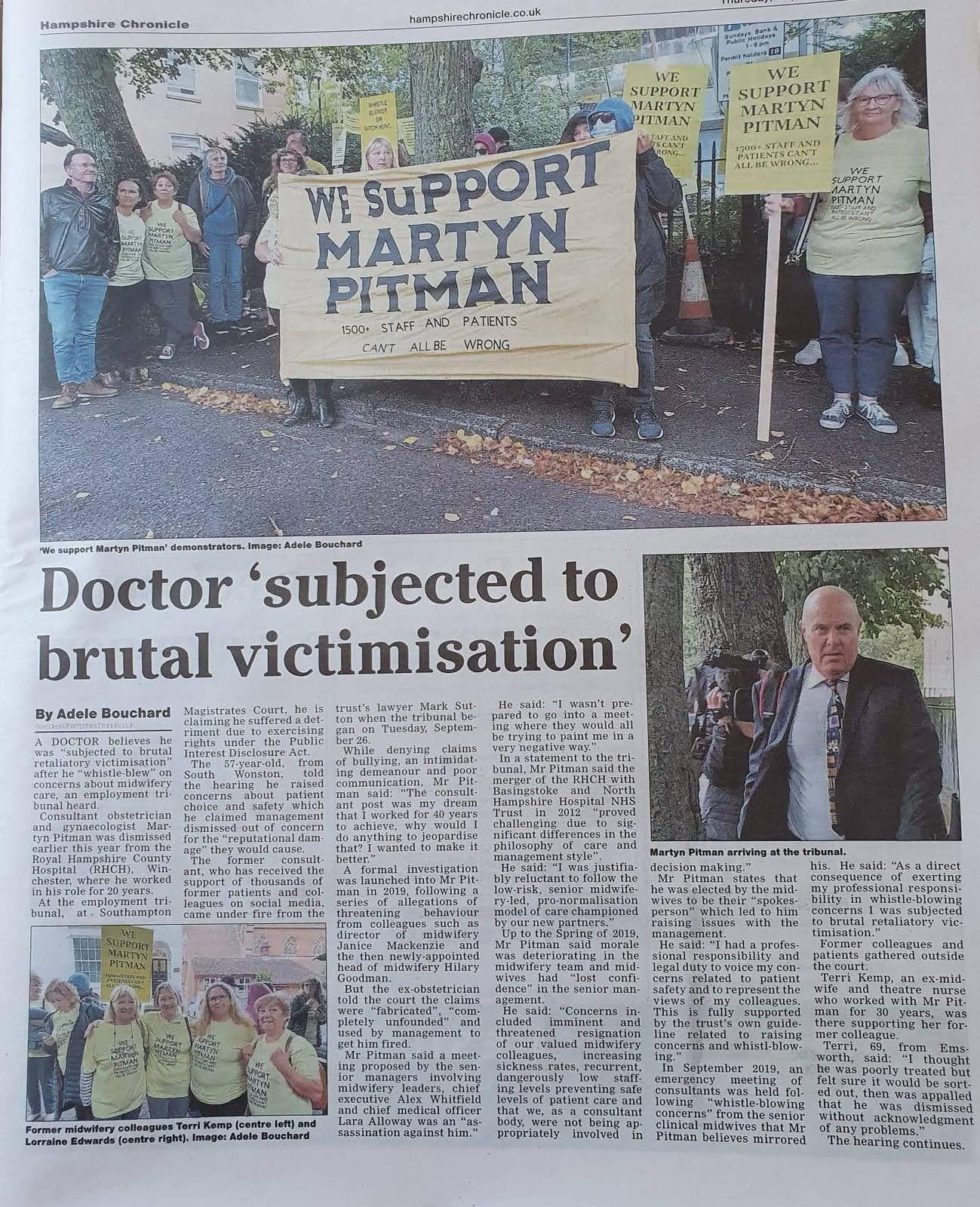The newspaper page, from the Hampshire Chronicle, features a detailed account of a protest supporting Dr. Mark Teon Pittman who is depicted in the article as being subject to brutal victimization. The top half of the page showcases a large photograph of a crowd holding yellow picket signs that read, "We support Mark Teon Pittman, 1,500+ staff and patients can't all be wrong." Among the crowd, many women are seen wearing yellow shirts with the same supportive message. In the bottom half of the page, the article includes additional photographs, including one of Dr. Pittman, a white bald man in a black suit and white shirt, preparing for court, and another of the protesting crowd. The article itself is by Adele Bucard and provides in-depth coverage of the events surrounding Dr. Pittman's circumstances.